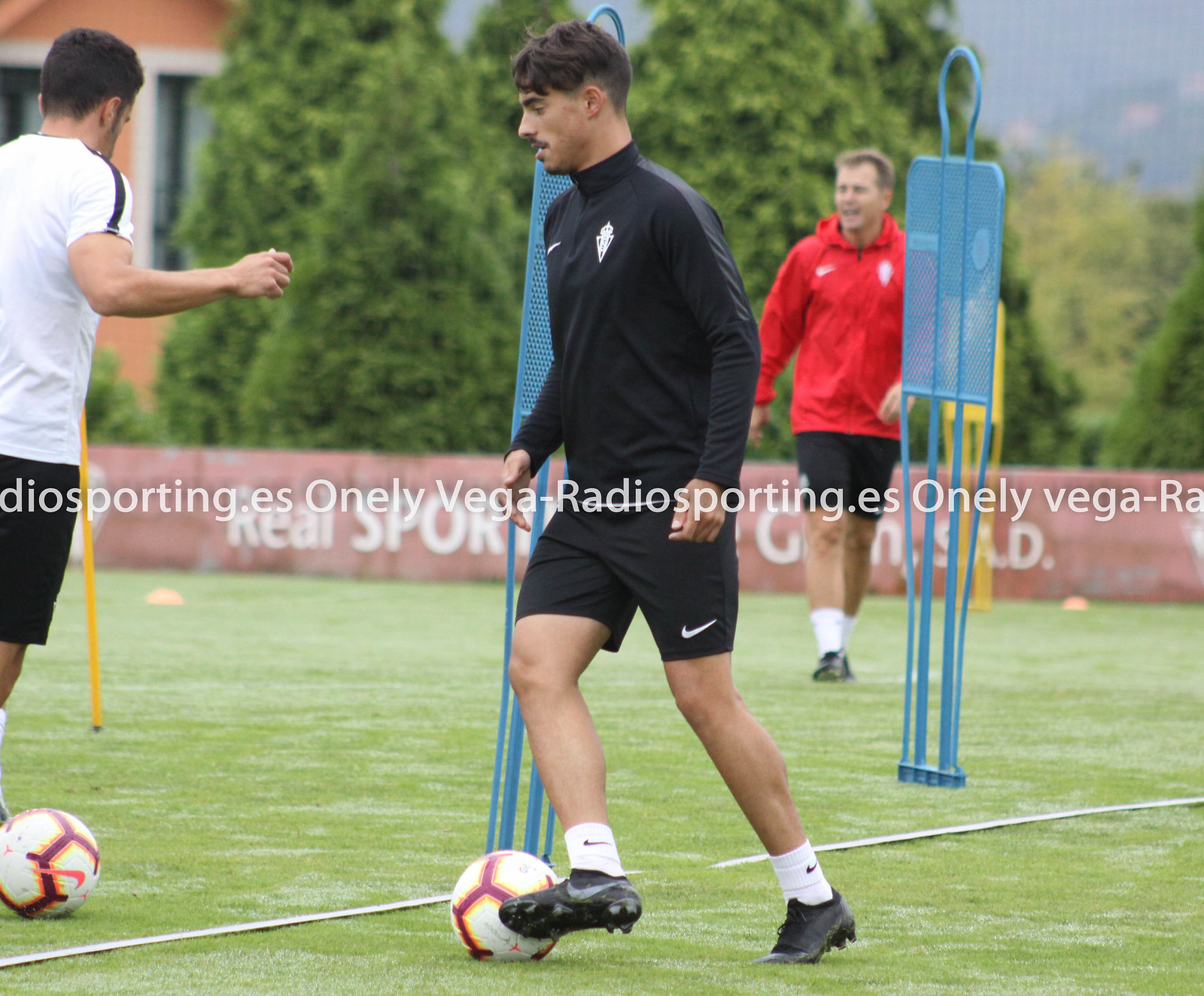In this detailed photo, three men are practicing soccer on a lush green field. The man on the far left, partially cut off by the edge of the picture, is wearing a white t-shirt and black shorts, with a ball near his leg. In the center, another man stands out as he runs and kicks a ball; he is dressed in a black long-sleeve shirt, black Nike shorts, white Nike socks, and black Nike soccer cleats. His short hair is clearly visible. Slightly to the right and further behind him, a third man in a red jacket, black shorts, white socks, and black shoes is walking towards the others. The field features two blue metal objects resembling human silhouettes, probably for dribbling practice. In the background, a fence with partial wording “Real Sport” is visible. Beyond the fence, green trees and a blue sky frame the scene, while a peach-colored building with windows is situated in the far left corner.